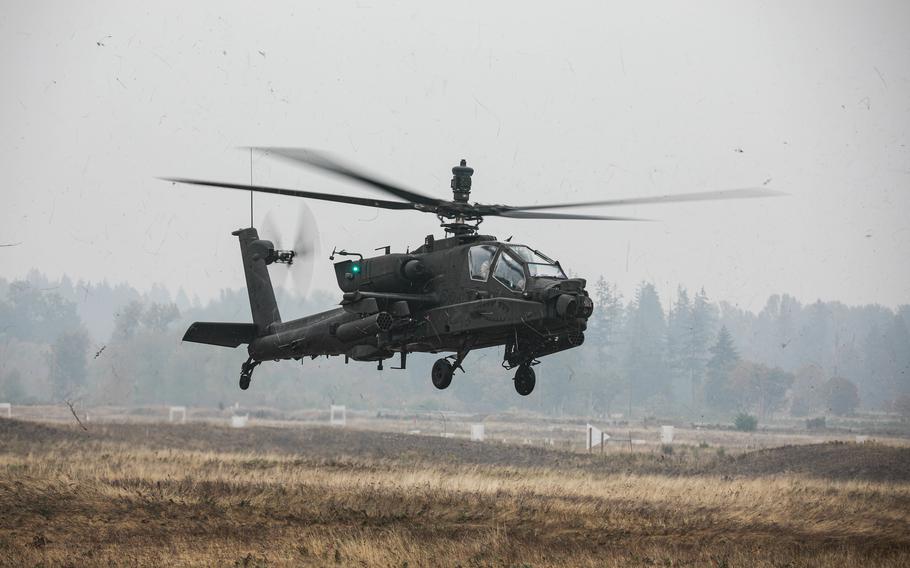In this detailed photograph, an AH-64D Apache Army helicopter is captured in mid-flight, hovering just above a vast, partially burned field. The helicopter, painted in a dark gray or black color, features a distinctive large disc atop its main rotor, which is a millimeter-wave radar attachment specific to this model. Both the main and tail rotors are in motion, their spinning blades appearing as a blur in the image. The aircraft's landing gear includes three wheels – two at the front and one at the rear. A subtle green light is visible on the helicopter's side, and the pilot can be seen in the cockpit. Below, the field is a patchwork of yellow and black, hinting at a landscape affected by either seasonal change or a recent fire. Surrounding the field is a stretch of tall trees, their form softened by a mist that envelops the area, suggesting a foggy day. Above the trees, the sky is a uniform gray, enhancing the moody and somewhat ominous atmosphere of the scene. In the distant background, white targets and possible remnants of an obstacle course further indicate that this is an Army training ground.